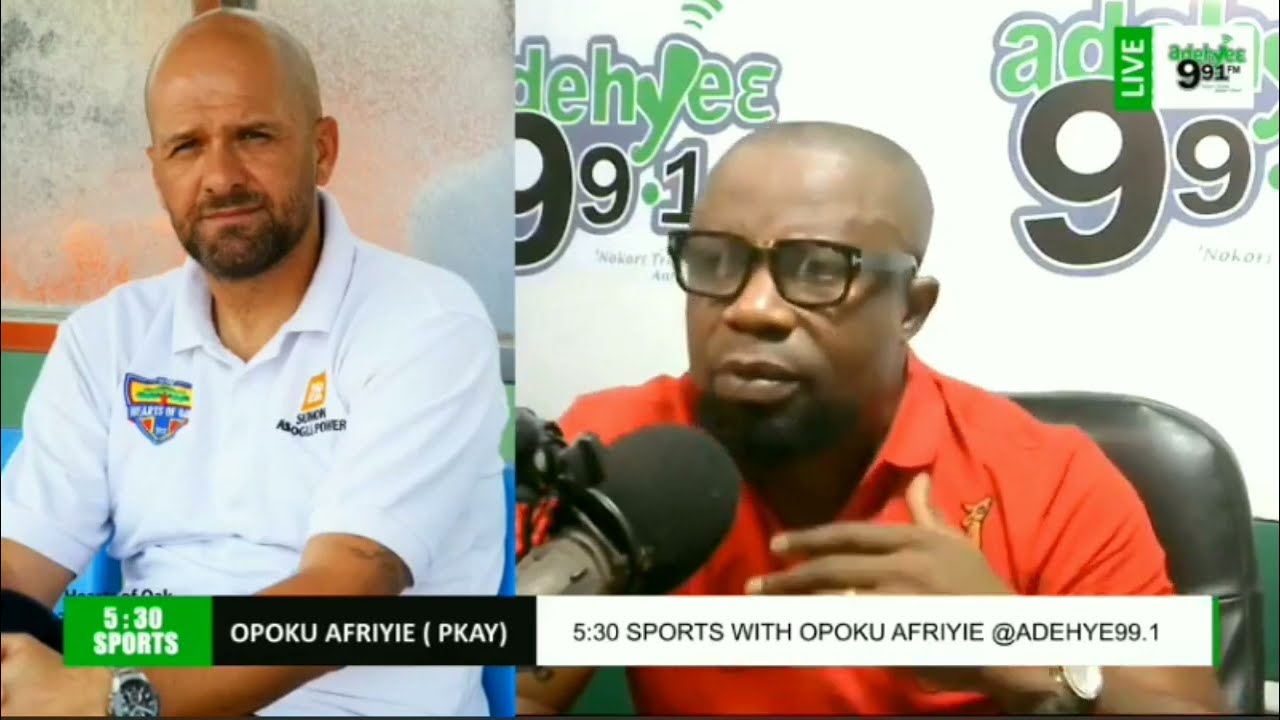The image is a wide rectangular screenshot of a video, depicting a split-screen broadcast. On the right side, there is a black male radio host with black-framed glasses, wearing a red short-sleeved collared T-shirt, and sitting in a black chair. He has a thin beard on his chin and is positioned in a radio station studio, speaking into a black microphone. Behind him, a wall displays the station's logo, "Adihe 99.1." On the left side, there is a white male in a white polo shirt featuring two logos. He is bald, with a thin black mustache and beard, and appears to be making a serious expression. In the upper right-hand corner of the image, the word "LIVE" is displayed horizontally, along with "Adihe 99.1." At the bottom of the screen, a series of bars provide additional information. The first green and black bar with white text reads "530 Sports; Opoku Afri PK," followed by a white bar with "530 Sports with Opoku Afri at Adihe 99.1" in black text.